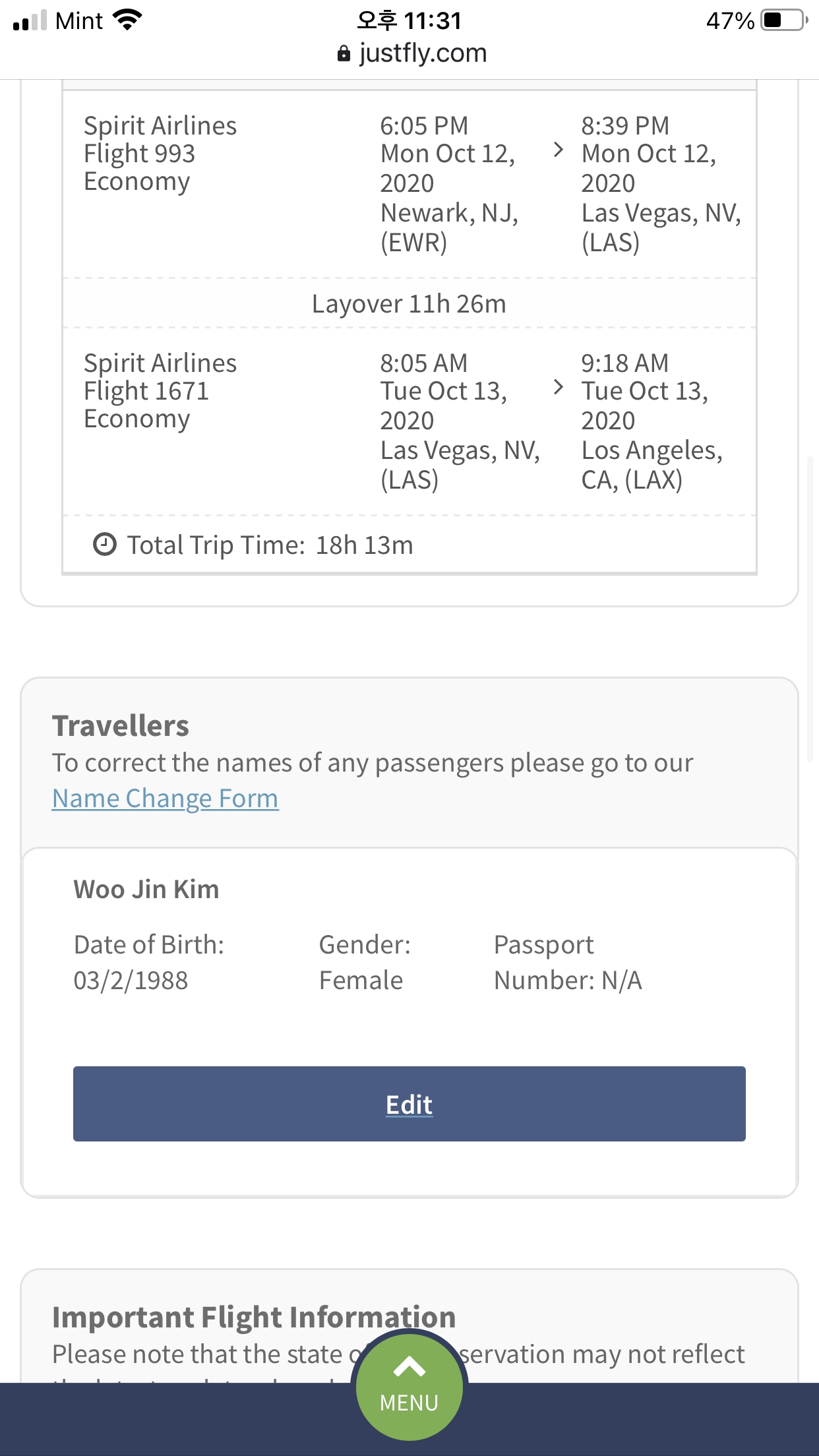The image is a screenshot from someone's cell phone displaying detailed information about booking an airline ticket. To the left of the screen, the signal bars indicate two out of four bars for the carrier signal, labeled as "Mint," followed by a Wi-Fi symbol showing full connectivity with four bars. Adjacent to this is oriental lettering and the time "11:31." Proceeding below, a small black padlock symbol and "JustFly.com" are visible. On the far right, the battery status is at 47% with a corresponding symbol.

The main content shows a booking for Spirit Airlines, flight 993, in Economy class, departing from Newark, New Jersey (EWR) at 6:05 p.m. on Monday, October 12, 2020, and arriving in Las Vegas, Nevada (LAS) at 8:39 p.m. the same day. The layover duration is listed as 11 hours and 26 minutes. 

The return flight details are for Spirit Airlines, flight 1671, also in Economy class, departing Las Vegas, Nevada (LAS) at 8:05 a.m. on Tuesday, October 13, 2020, and arriving in Los Angeles, California (LAX) at 9:18 a.m. on the same day. The total trip duration amounts to 18 hours and 13 minutes.

Following this, there's an instruction for travelers to correct passenger names via a "name change form," indicated as an underlined blue hyperlink. The traveler information includes Woojin Kim, with a date of birth of March 2, 1988, gender marked as female, and passport number as "NA". A blue rectangle labeled "EDIT" appears below this.

Lastly, the section titled "Important Flight Information" includes a message about the state of the reservation potentially not reflecting, though most of this text remains obscured by a dark blue horizontal rectangle with a green circle and an upward-pointing white arrow, along with the word "menu."

The screenshot indicates that the individual, Woojin Kim, is finalizing plans to purchase a ticket for the outlined flight itinerary.